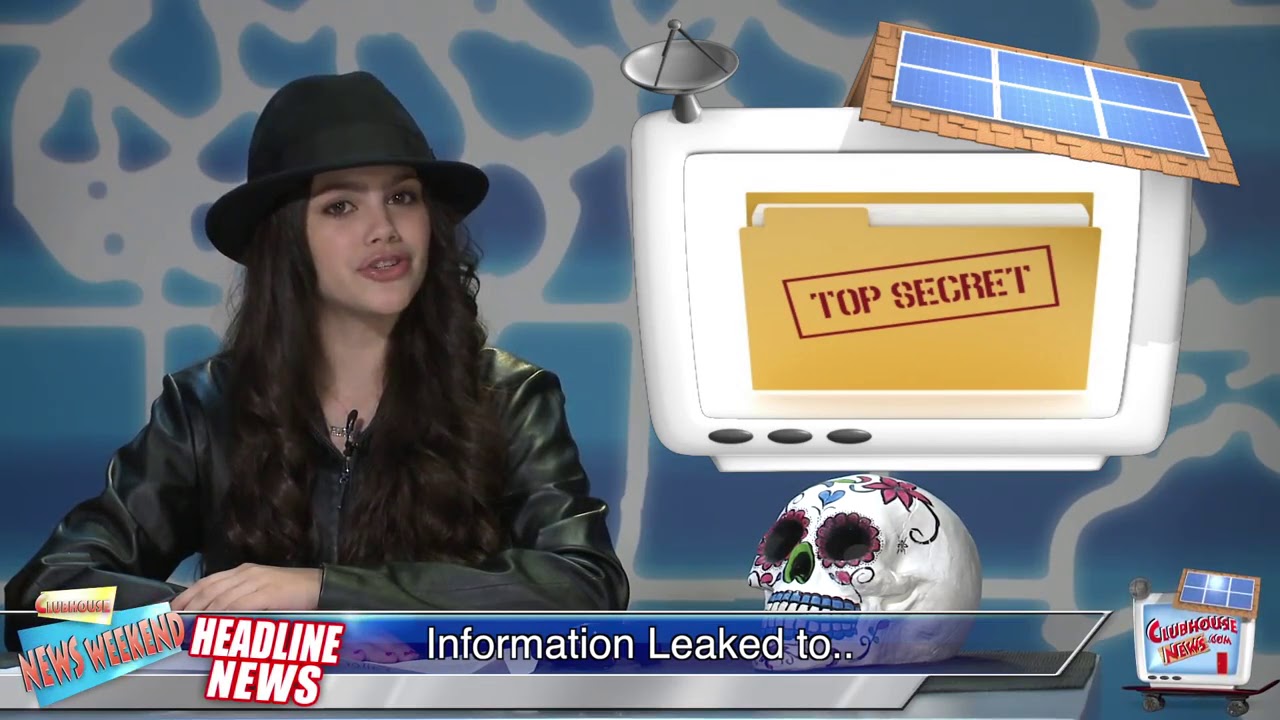The image is a horizontal, rectangular photograph that appears to be a spoof on a television news broadcast, possibly aimed at children. It features a young woman with lighter skin and long, curly black hair, wearing a black leather jacket and a black bowler hat. She sits on the left side of the image, behind a desk with a silver frame and a black top. The background is a blue wall adorned with white abstract lines and shapes. To her right sits a white sugar skull decorated in bright colors: pink flowers around the eyes, green on the nose, and blue accents around the teeth, with additional floral designs in pink and green on the head. Positioned near the woman is a stylized drawing of a white TV screen with a six-pane window that displays a file folder labeled "Top Secret." It features a gray satellite dish on the left and a tiled roof with solar panels on the right. At the bottom of the image, a text banner displays multiple headlines in various colors and shapes: "Headline News" in white letters outlined in red, "Information Leaked To" in white letters within a blue streamer, "News Weekend" in red letters within a blue square, and a partially obscured "clubhousenews.com."